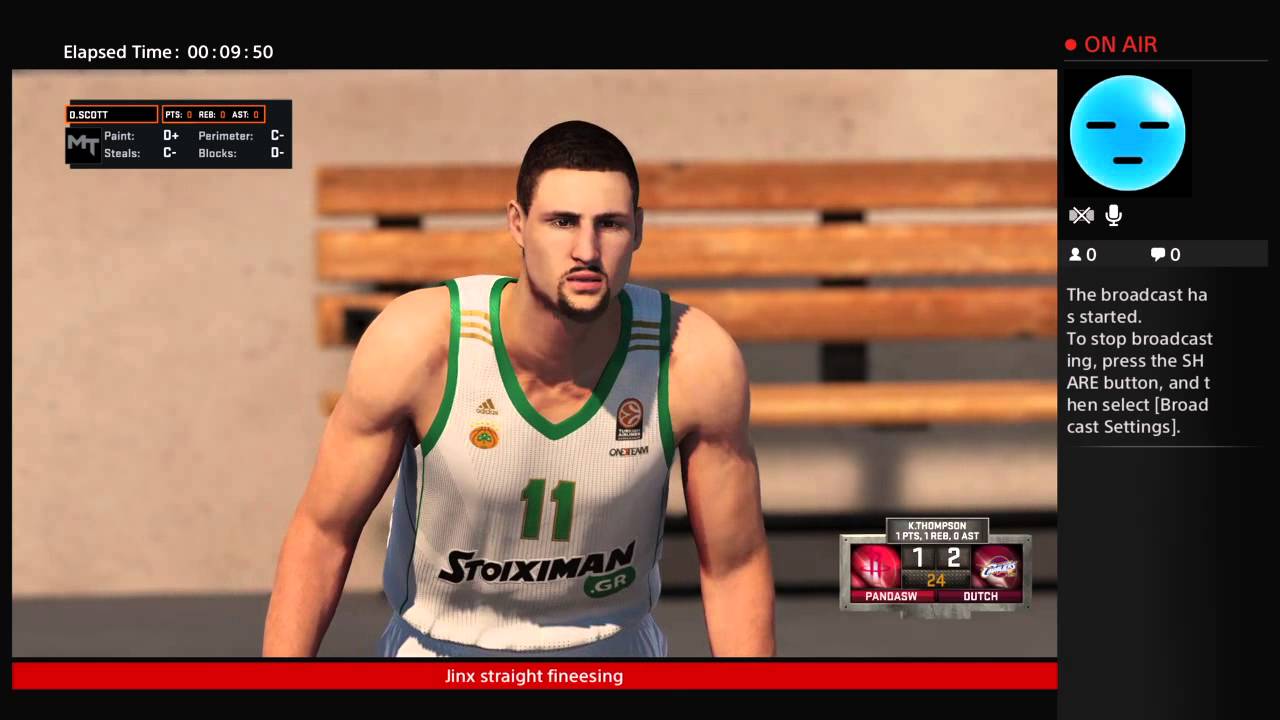The image features a screen capture from a digital basketball game, set against a black background. In the upper left-hand corner, there is a white timer displaying "Elapsed Time: 00:00:09:50," accompanied by a red bullet point and the text "On Air" in red. 

At the center of the image is a player with close-cropped dark hair and facial hair, wearing a white tank top with green armbands. The neckline of the tank top also has green detailing. The player's jersey features several logos and displays the number 11, with "Stokesman.gr" emblazoned on the chest. The player appears muscular and is positioned in front of a bench, with a tan wall behind and a gray floor beneath him.

A red bar runs along the bottom of the image, overlaying the player, with the text "Jinx straight finessing." In the upper left-hand corner, there is a black box containing two orange rectangles. The left rectangle reads "Zero Scott," while the right one says "PTS," though the point value is not legible. The acronym "R.E.D." is also visible near these details.